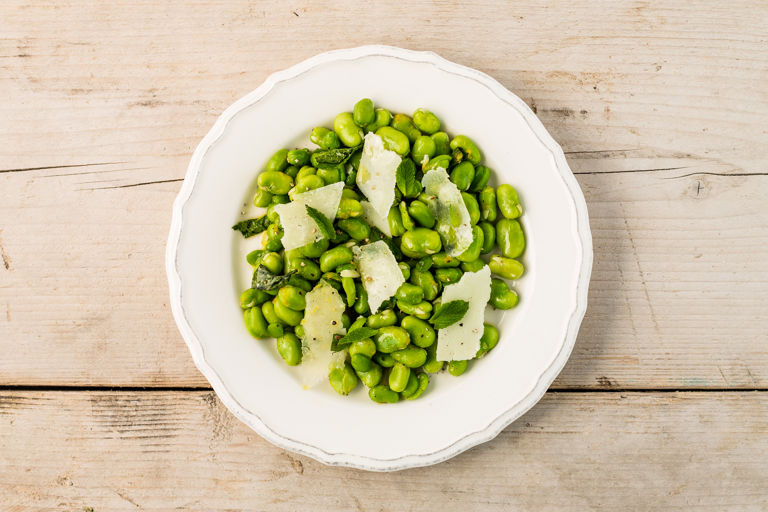The image captures a bright, colorful scene of a simple yet elegant meal placed on a wooden table, which shows evidence of natural cracks and light staining across multiple pieces of wood. The focal point is a white, scalloped plate with a decorative border that becomes darker towards the edges. The plate is filled with shelled edamame beans, which are slightly shiny, suggesting they are coated in melted butter. Sprinkled on top of the beans are seven pieces of grated Parmigiano-Reggiano, adding a rich texture and flavor. The dish is further seasoned with sporadic flecks of cracked pepper, enhancing the visual appeal and taste of this vibrant and appetizing meal. The good lighting in the image accentuates the greens of the edamame and the yellows of the cheese, making the dish appear fresh and delicious.